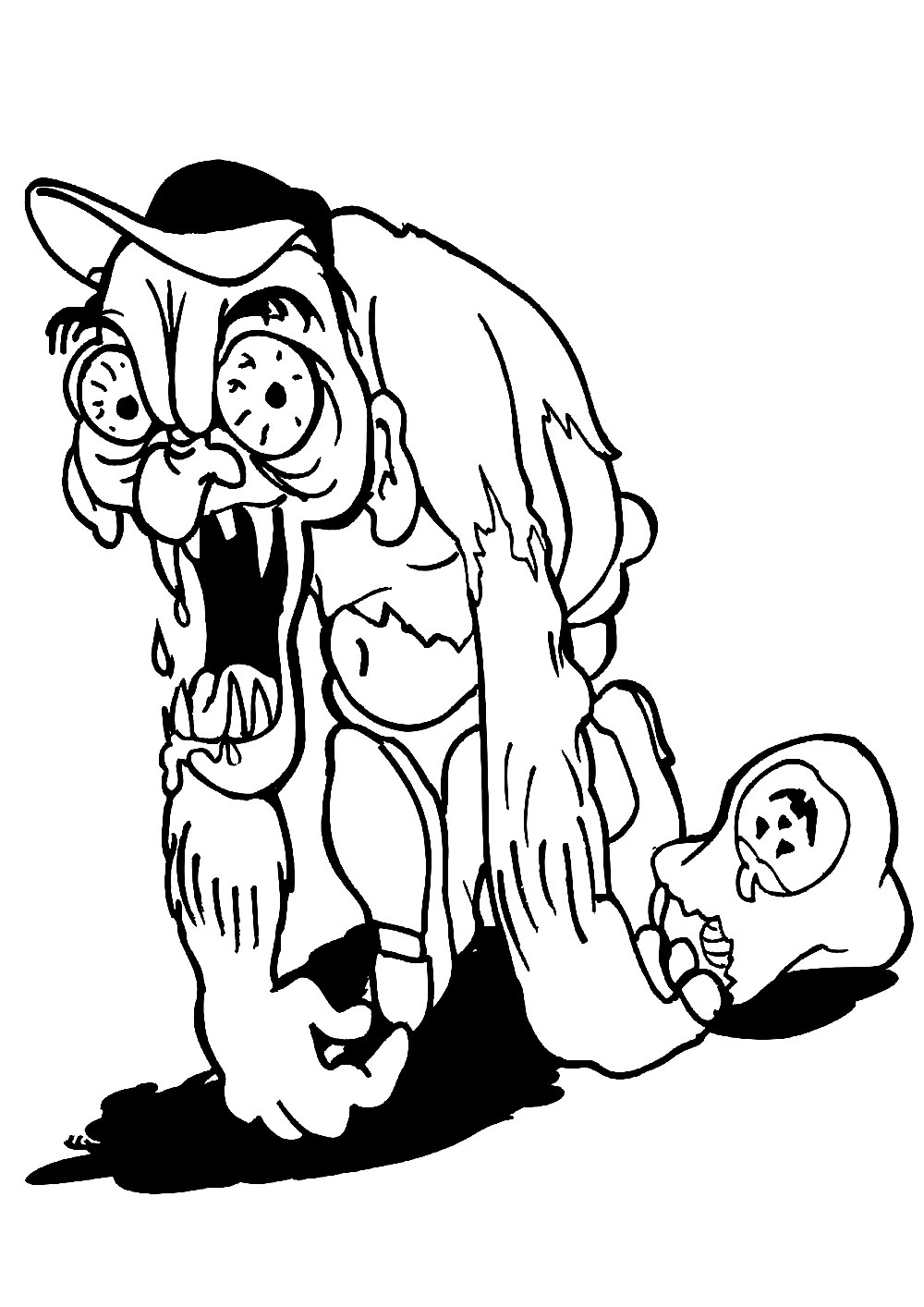The image is a detailed black and white illustration of a menacing zombie-like creature, drawn with a horror-themed style. The creature is centrally placed and occupies most of the image, emphasizing its haunting presence against a stark white background. 

This monster is depicted in a hunched posture, dragging its long, muscly arms on the ground in front of it. Its right hand clutches a trick-or-treat bag adorned with a jack-o'-lantern, indicating a Halloween setting. The creature’s facial features are grotesque: it has large, round, bloodshot eyes with pronounced squiggles to highlight their eerie appearance, and its sagging, furrowed forehead is topped with bushy eyebrows. It has a misshapen nose, large droopy ears, and a cavernous mouth filled with sharp, fang-like teeth, from which drool drips menacingly. 

The zombie wears a tattered shirt with jagged edges, exposing its wrinkled belly, and simple pants, though clothing details are minimal. It sports a black baseball cap with a white brim, adding a peculiar, almost ironic touch to its terrifying appearance. The overall style is minimalist, with an absence of shading and a focus on bold, defining lines, making it suitable for a coloring book or similar artwork.